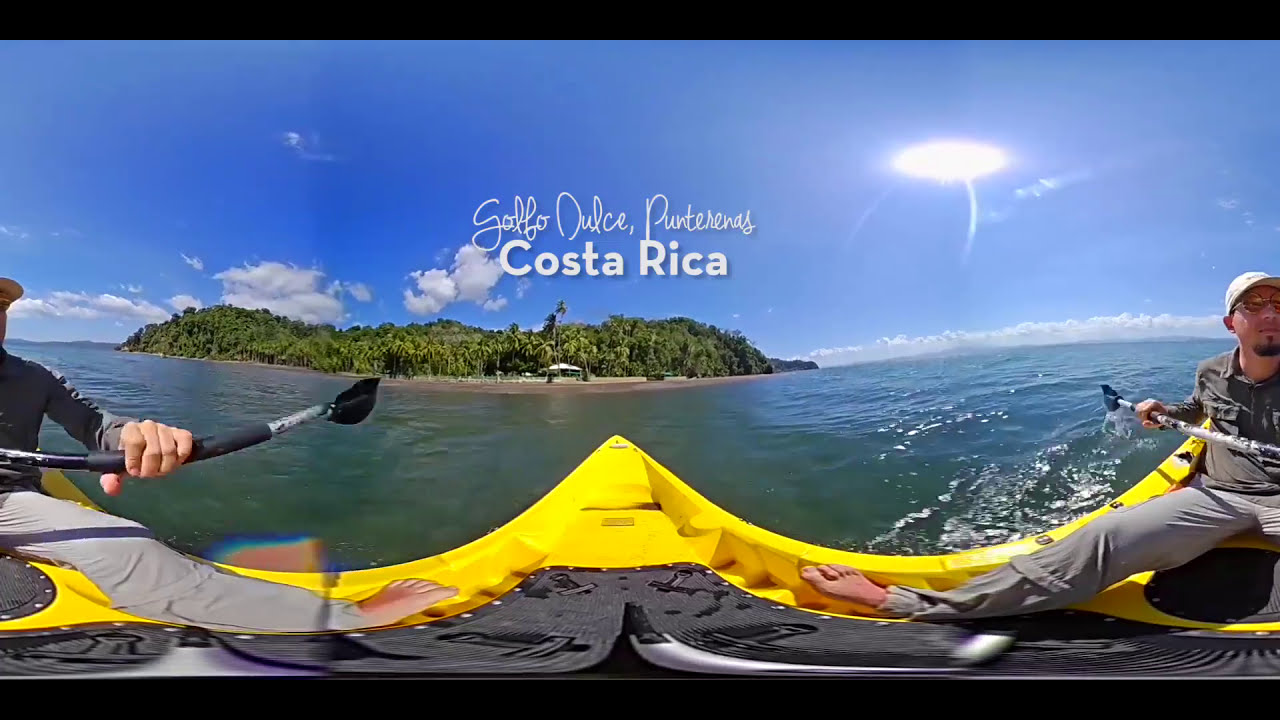This is a panoramic photograph taken mid to late afternoon in Costa Rica, focusing on a yellow canoe with black accents. The center of the image features script text in white, reading "Gulfo Dulce Punta Neres," with bold white text below saying "Costa Rica." The scene captures a man with glasses, a white hat, a dark gray shirt, and light gray pants, barefoot and paddling. Due to the panoramic shot, the image appears to have two people, but it is actually the same person duplicated. The canoe is navigating clear, greenish-blue waters towards a lush island with dense green trees and a small, white structure. The sky is a stunning dark blue, with a large sun descending and white puffy clouds in the distance.